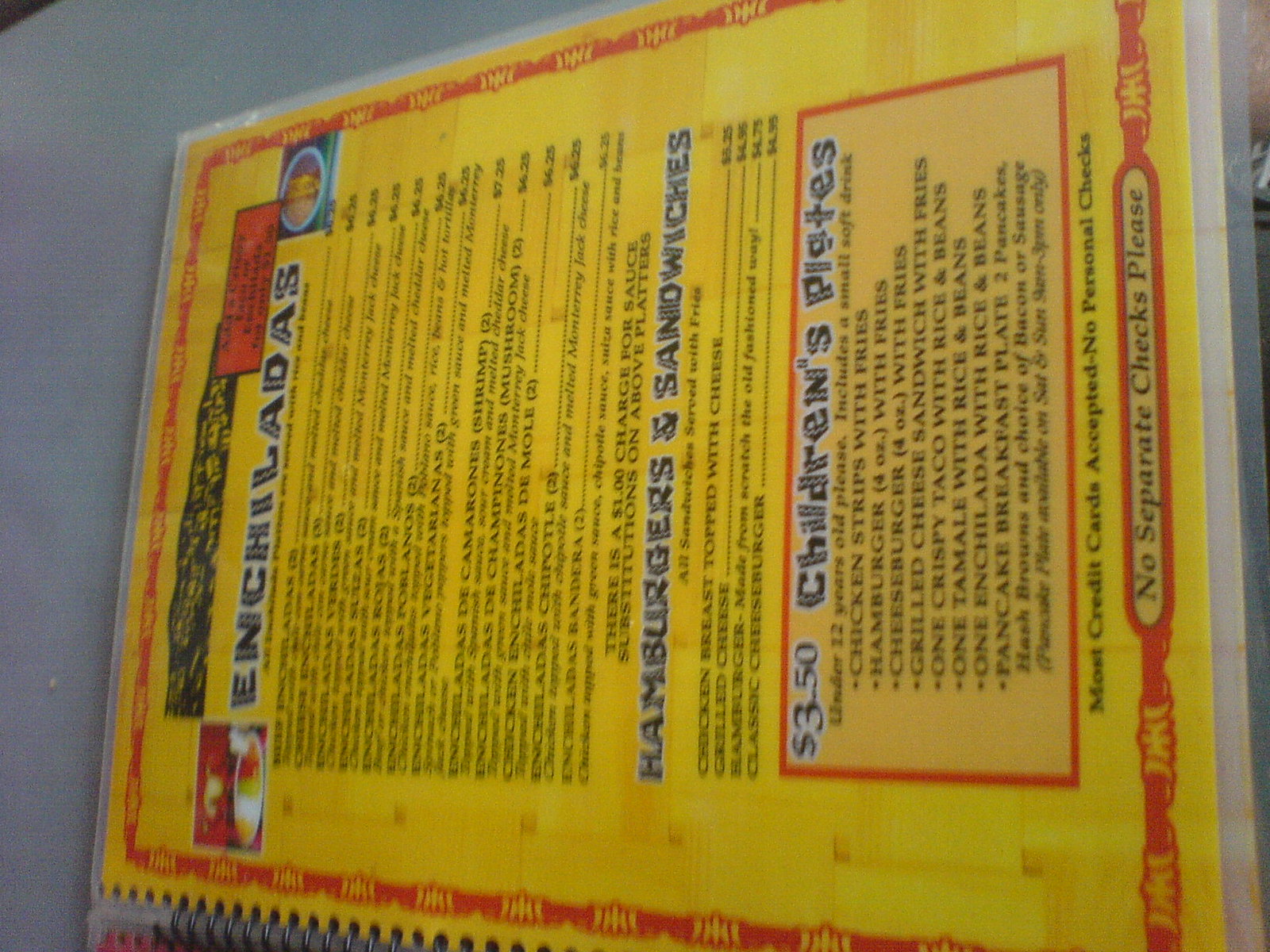The image displays what appears to be a menu from a Latin restaurant, captured at a slight angle which makes it somewhat difficult to read. The menu has a yellowish-orange background with a festive black text header at the top, prominently displaying the word "Enchiladas". Flanking the text on both sides are small images of dishes: the left one featuring a colorful plate with red, green, white, and yellow elements, and the right one showcasing a bowl containing a yellowish dish. Below the header, there is an extensive list of over 15 different dishes. 

Additionally, sections for "Hamburgers and Sandwiches" and "Children's Plates" are visible. The 'Children's Plates' section, enclosed in a box, lists items such as chicken strips, hamburgers, cheeseburgers, grilled cheese, and one crispy taco for $3.50. The entire menu is bordered by a reddish-orange frame and appears to be laminated. At the top of the menu, there is a black strip adorned with small yellow shapes, adding to the menu's festive Latin aesthetic.